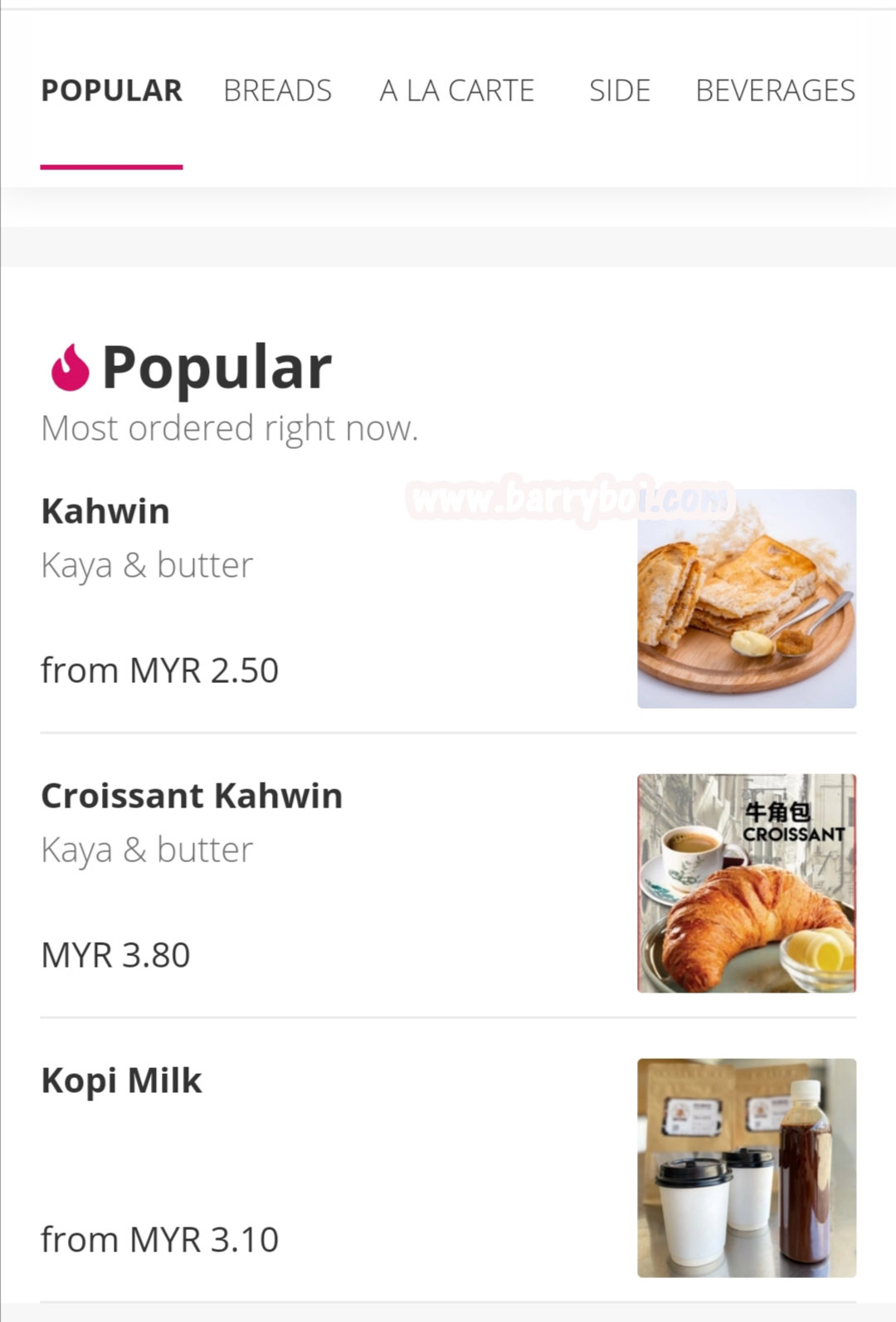This image is a screenshot from a website or mobile application, cropped to showcase a specific section of information. A faint watermark reading "www.barryboy.com" runs across the screen, outlined in baby pink. The header section of the screenshot features navigational menu buttons, with the "Popular" tab currently selected. Other available menu options include "Breads à la Carte," "Sides," and "Beverages." This setup suggests the platform allows for online ordering, likely for a restaurant or takeaway service.

Within the "Popular" tab, there are three highlighted menu items, signified by a bright pink fire icon and the tagline "Most ordered right now." The top item is "Carwin, Kaya, and Butter," accompanied by a small thumbnail image. The second item is "Croissant Carwin," also shown with a small image. The third option is "Kopi Milk," depicted with a small image of two takeaway cups and a bottle. The prices are listed in MYR (Malaysian Ringgit), indicating the currency used is not English.